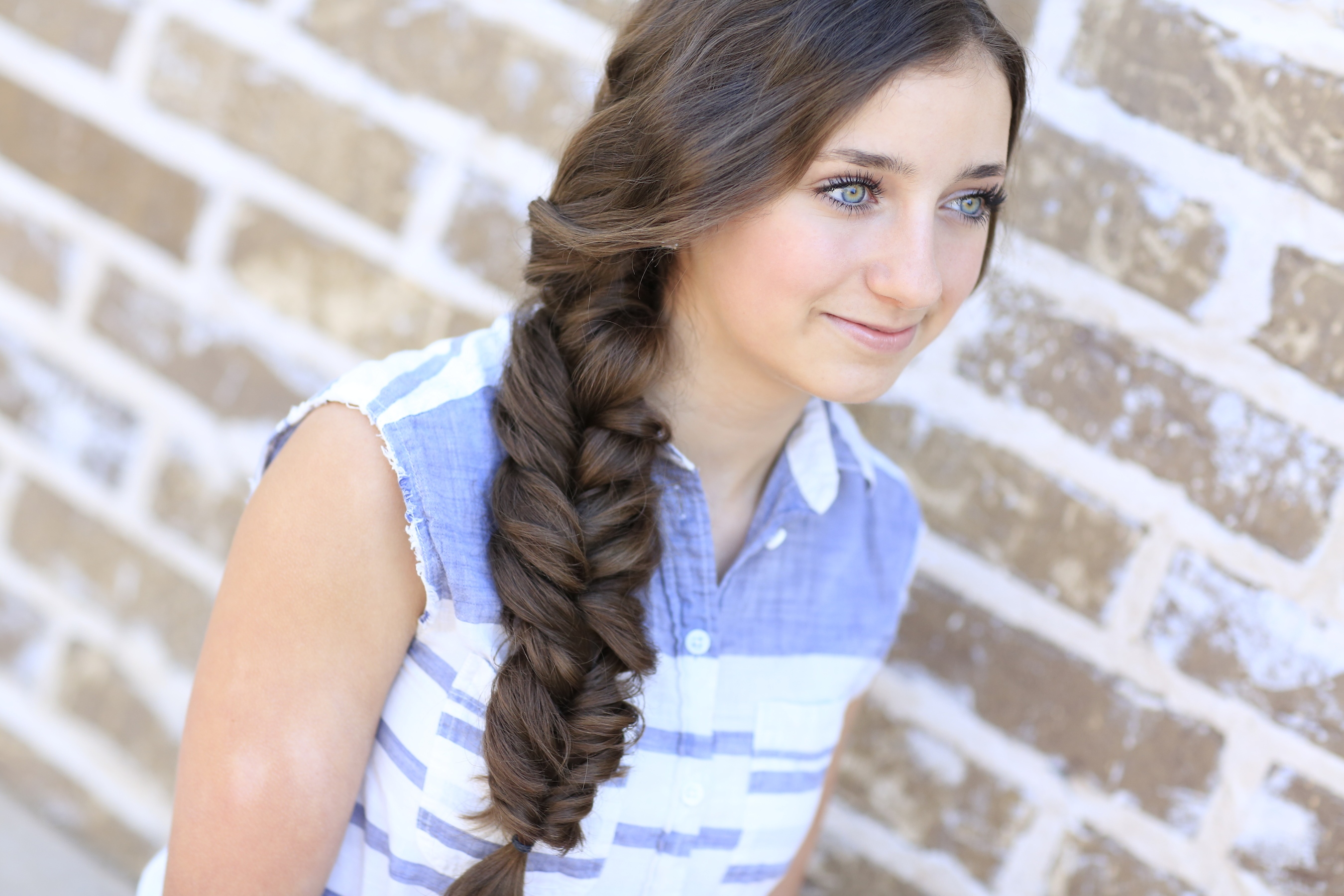The image depicts a young woman, likely around 18 years old, with long, brown hair that is neatly braided and draped over her right shoulder. Her hair is parted in the middle, and the braid extends from her neck down to just below her breast. She has striking eyes with a unique blend of blue and green hues, accentuated by black eyeliner. Her light pink lips and fair complexion give her a subtle, yet radiant appearance.

The woman is wearing a sleeveless, button-down shirt with a blue and white pattern. The top button of her shirt is unbuttoned, while the remaining buttons are secured, all of them white. The shirt features a design that includes stripes extending down the front and back, with a solid blue section around the shoulders.

She is standing against a reddish-brown brick wall, which is held together by conspicuous white cement. The wall has patches of white blotches, adding texture to the background. The photo is taken outdoors, as evidenced by the sunlight faintly visible in the background. The image captures her from the chest up, with her eyes, particularly their captivating blue tones, drawing significant attention. She appears to be gazing towards the right side of the image, adding a sense of contemplation to her expression.